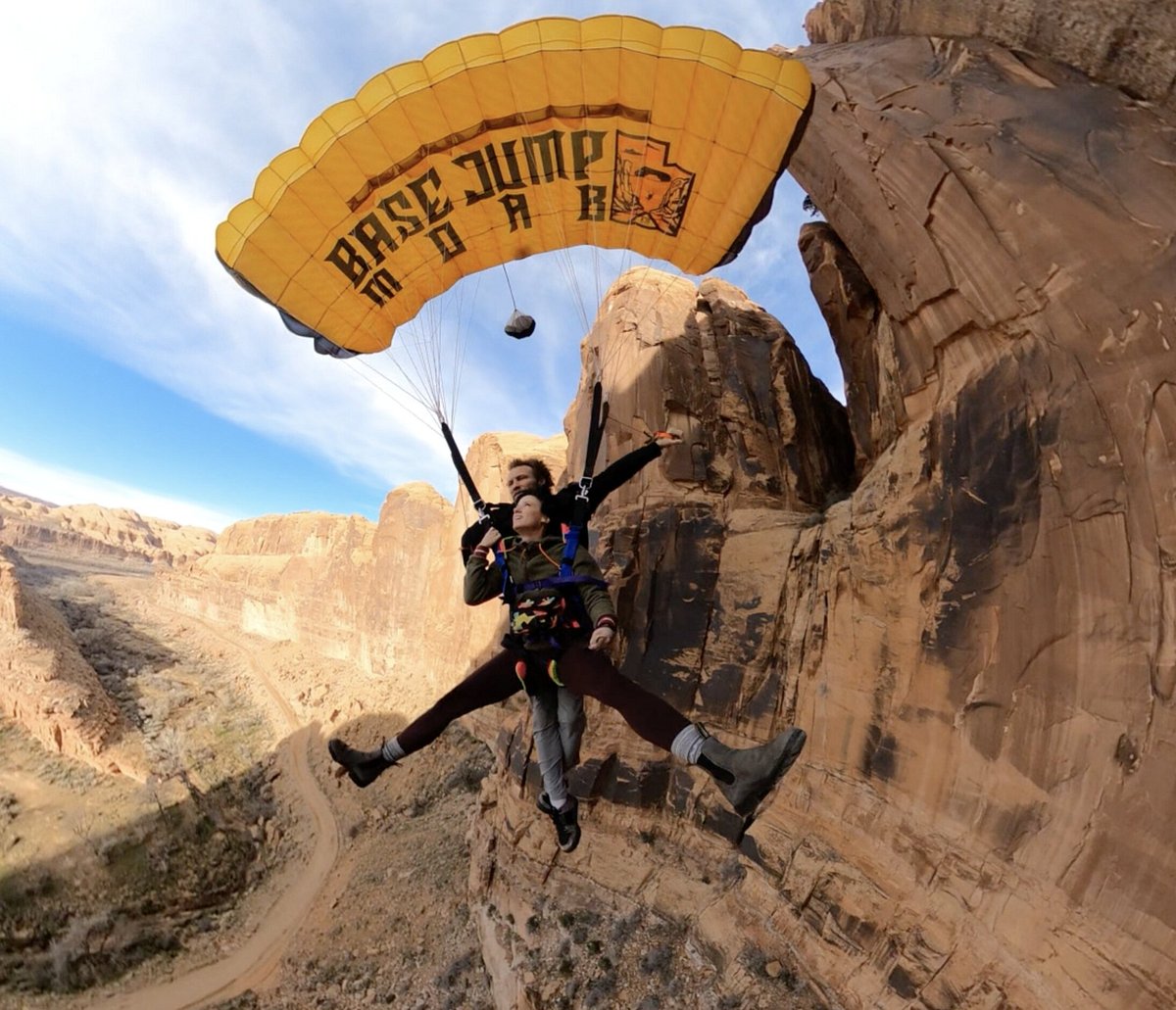This photograph captures a thrilling moment in a stunning canyon landscape, likely part of a national park with towering, reddish-beige rocky formations. The image centers on two adventure-seekers, a man and a woman, connected by a bright yellow parachute emblazoned with the text "BASE JUMP MOAB" in black letters alongside an orange symbol. The woman, strapped in front of the man, has her legs splayed wide in an "A" position, while the man behind her has his legs hanging straight down. Both are equipped with black straps and heavy boots. The scene suggests they have just leaped off a cliff, as they soar through the air descending gracefully amidst the rugged, barren rock formations below. Above, the sky is a brilliant blue, adorned with thin, wispy white clouds, adding to the dramatic and exhilarating atmosphere of their adventure.